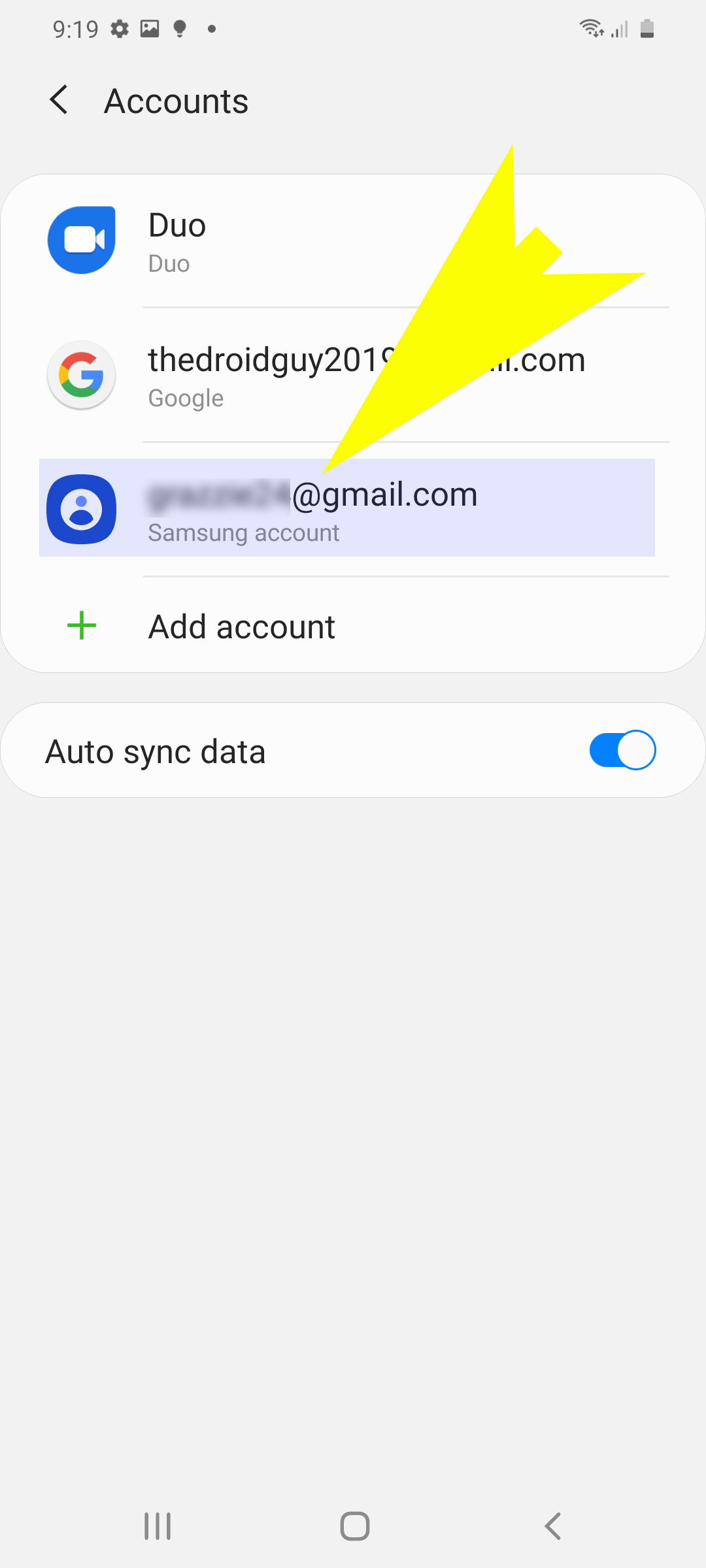The screenshot presents a smartphone display showcasing an "Accounts" settings page. The background is primarily grayish-white, with various selectable fields in shades of blue or white. At the top of the screen, the title "Accounts" is displayed alongside a back arrow for returning to the previous screen.

Beneath the title, there are three account windows:

1. The first window is labeled "Duo" and features a blue video icon.
2. The second window includes the Google account “Droid Guy 2019” accompanied by the colorful Google "G" logo.
3. The third window, which is highlighted in light blue, displays a grayed-out name with "gmail.com" indicating a Gmail account. This window also contains a small icon depicting a figure in a white circle bordered by a blue shape that is semi-rectangular, semi-circular, or oval. Superimposed above this selection is a large yellow arrow pointing directly at it.

Below these three windows, there is a fourth option titled "Add Account" with a green plus icon next to it. Further down, another window appears with a toggle button that is switched on, labeled "Auto Sync Data." 

The bottom of the screen contains a large gap followed by the primary navigation controls of the smartphone, including a reverse arrow, allowing the user to navigate back or perform other standard functions.